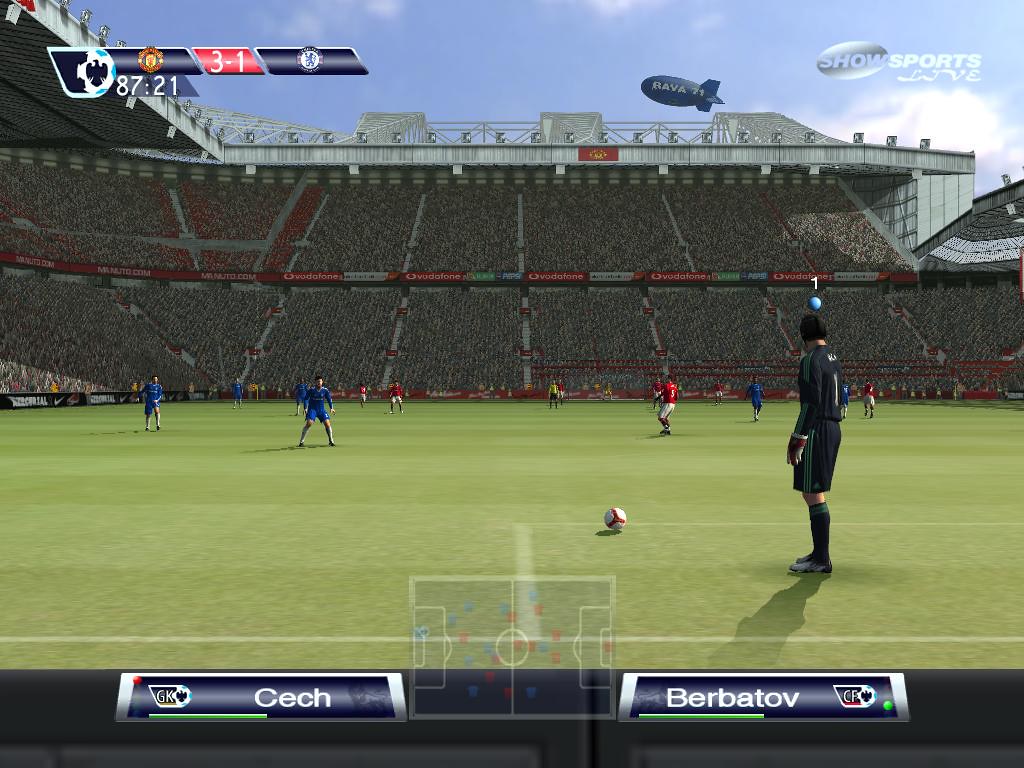This screenshot captures an intense moment from a soccer video game. The screen displays the scoreboard at the bottom left, showing "C-E-C-H" as one team's name, while the opposing team, "B-E-R-B-A-T-O-V," is listed on the right. Players on the field are creatively distinguished by their jerseys: some are dressed in black, others in blue, and a few in red and white. In the backdrop, individuals clad in yellow are visible, possibly game officials or additional players. The stands around the soccer field are packed with enthusiastic spectators, adding to the excitement of the match. High above, a bright blue sky with scattered clouds provides a picturesque setting, further enhanced by the presence of a blimp displaying some letters. In the top right corner, the text "Show Sports Live" in white marks the broadcast of this thrilling gameplay.